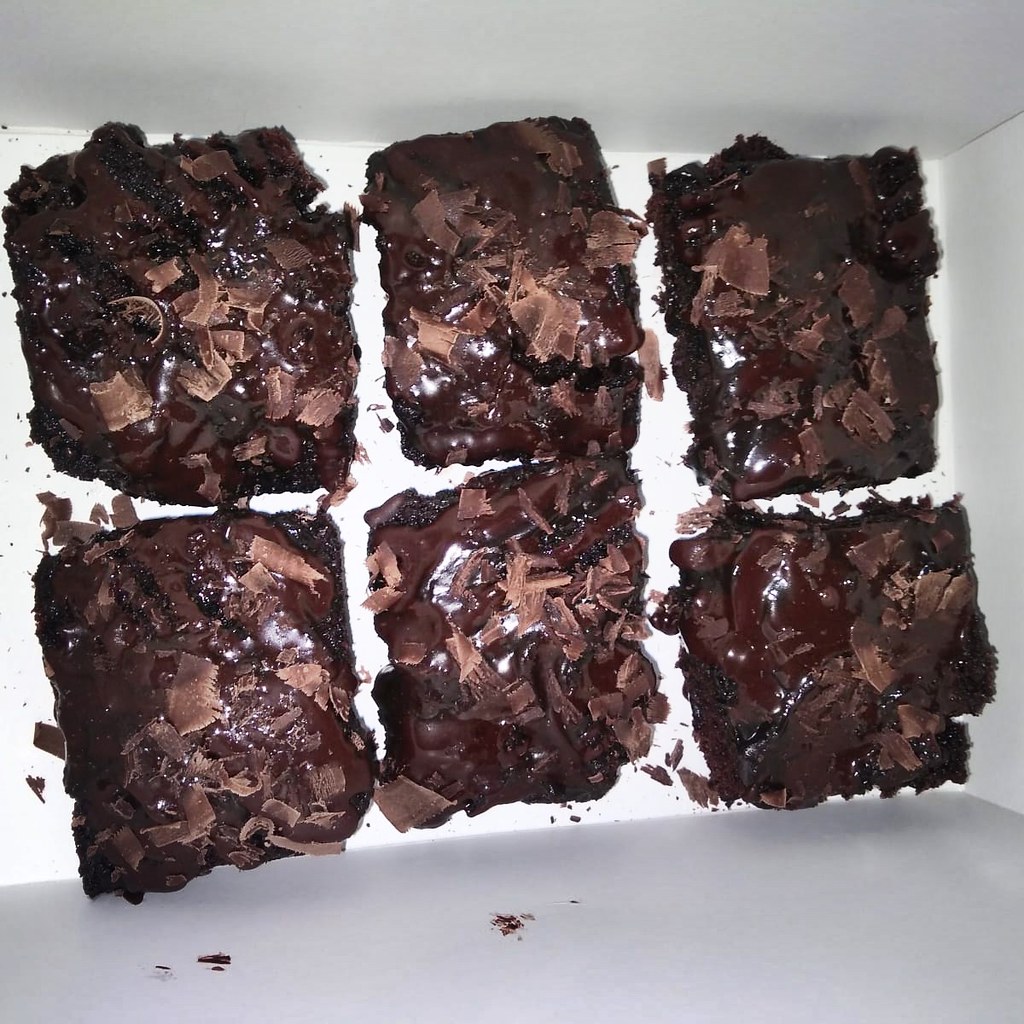This photograph provides a bird's eye view into a white cardboard box containing six deeply rich chocolate brownies, arranged in two rows of three. The brownies, cut into uneven square shapes with rough edges, showcase a slightly messy yet indulgent appearance. Each brownie is topped with a layer of lighter brown chocolate shavings, some of which have fallen to the bottom of the box. Additionally, two smudges of chocolate are visible on the interior walls of the box, adding to the overall impression of a deliciously messy treat. The image captures the decadent and imperfectly charming nature of these chocolatey delights, ready to be enjoyed by an eager recipient.